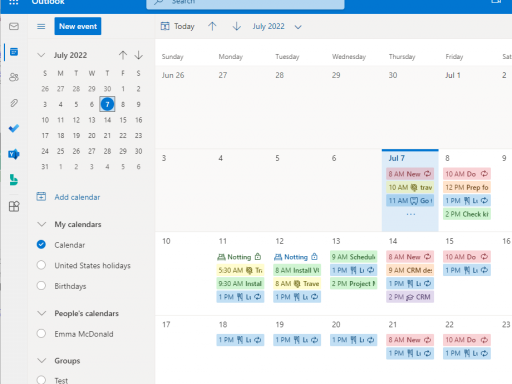This screenshot displays a Microsoft Outlook calendar interface, likely captured on a laptop, given its landscape orientation. In the upper left corner, the light blue of the Outlook tab is visible. At the top center is a search bar. Just below, icons are arrayed: a small envelope, a three-line menu bar, and a prominent blue "New Event" button. 

The current date, marked as July 22 with a dropdown arrow, resides adjacent to navigation arrows for moving through dates. On the left sidebar, July 7th, 2022 is highlighted, indicating active organization starting from this date. The calendar shows a structured list of events: 

- **July 7th:**
  - 8:00 AM: "new" (text only)
  - 10:00 AM: "travel" (with a travel-related emoji)
  - 11:00 AM: Appears to be a dentist appointment (dentist-related emoji)

- **July 8th:**
  - 10:00 AM: "due"
  - 12:00 PM: "prep"
  - 1:00 PM: Appearing to be lunchtime (fork and knife emoji)
  - 2:00 PM: "check"

This pattern of detailed planning continues throughout the weekdays, reflecting a meticulous and organized schedule. Notably, for the 18th, 19th, and 20th, the 1:00 PM slot is consistently marked with a fork and knife emoji, likely denoting lunchtime, integrated into their daily routine.